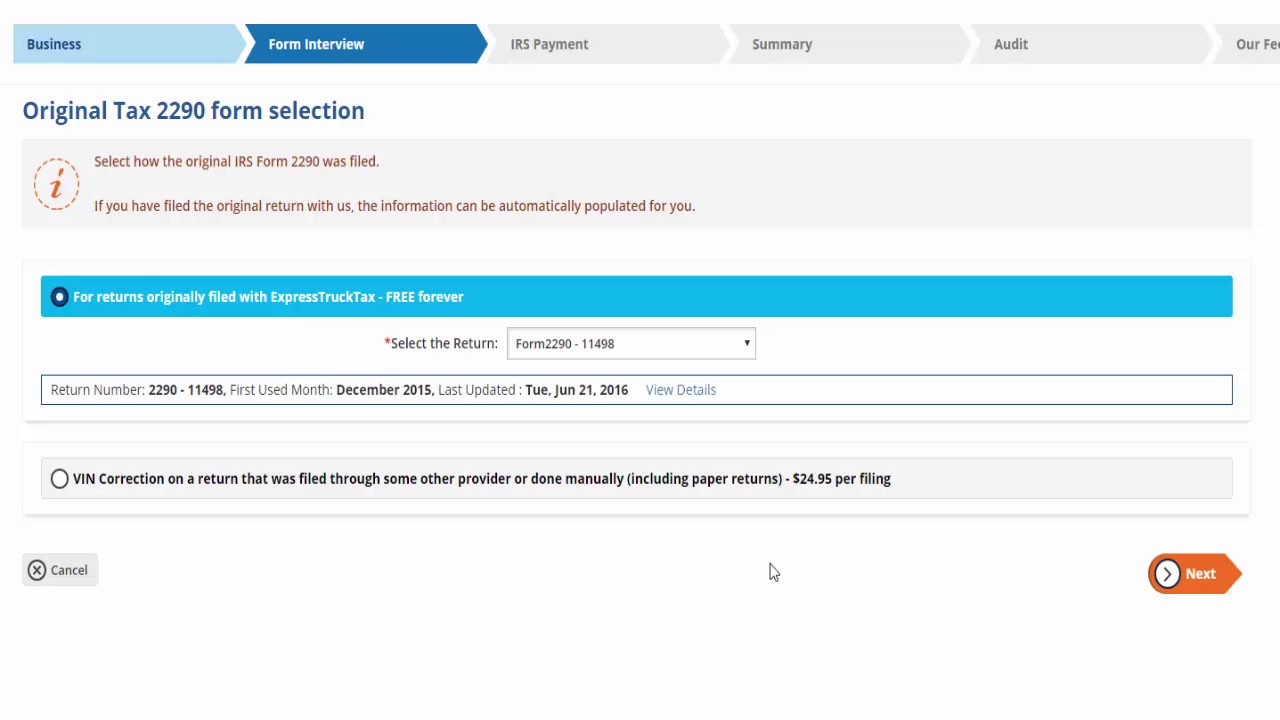This image displays a webpage designed for selecting an original IRS Form 2290. At the top of the page, wide arrows interlock, indicating a multi-step process. The steps identified in these arrows are, from left to right: "Business", "Form Interview", "IRS Payment", "Summary", "Adopt", "Our", with the last step cut off and not visible in the image.

Below the arrows, a prominent header in red reads, "Original Tax Form 2290 Selection." Just under this header, additional text instructs the user to select how the original IRS Form 2290 was filed, also in red: "Select how the original IRS form 2290 was filed. If you have filed the original return with us, the information can be automatically populated for you."

To the side, there is a cursive lowercase letter "i" surrounded by a dotted circular line, in a reddish-orange hue, likely indicating additional informational resources.

Continuing down the page, there is a blue rectangle with the text, "For returns originally filed with Express Truck Tax-Free Forever," accompanied by a clickable dot. The page concludes with a red "Next" button located at the bottom right corner, guiding the user to proceed.